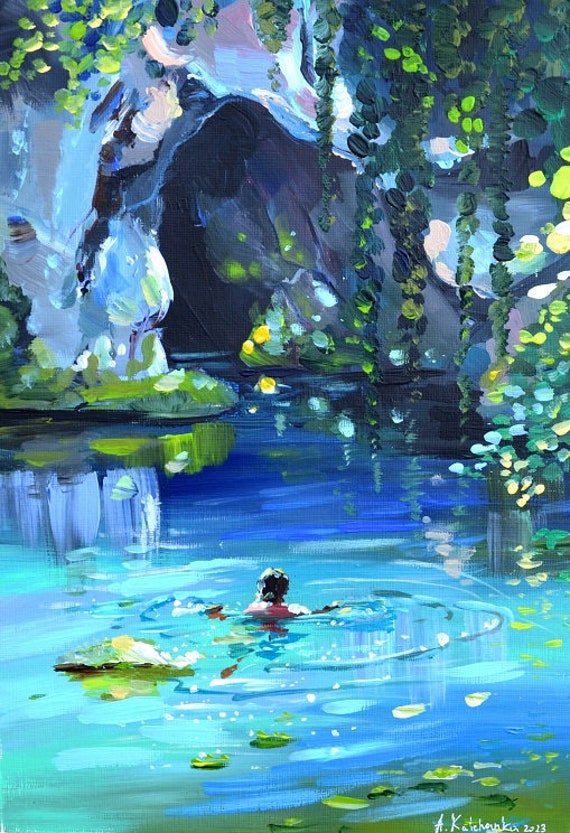The image is a detailed painting of a serene pond set deep in a lush forest, with dominant hues of blue and green. The water is a striking, crystal-like blue with a deeper shade towards the cave-like stone arch that forms a natural bridge over the pond. A lone swimmer, seemingly a female, is depicted from behind, with only their head and shoulders visible as they swim under the stone arch. The scene is surrounded by overhanging plants, including ivy and green lotus leaves, which add to the natural beauty of the setting. The reflections in the water are meticulously painted, creating small waves that radiate from the swimmer. This piece, signed by an artist with the initial "A" and dated 2013, showcases the tranquil yet vibrant environment of this picturesque pond, blending elements of sparse human presence and untamed nature.